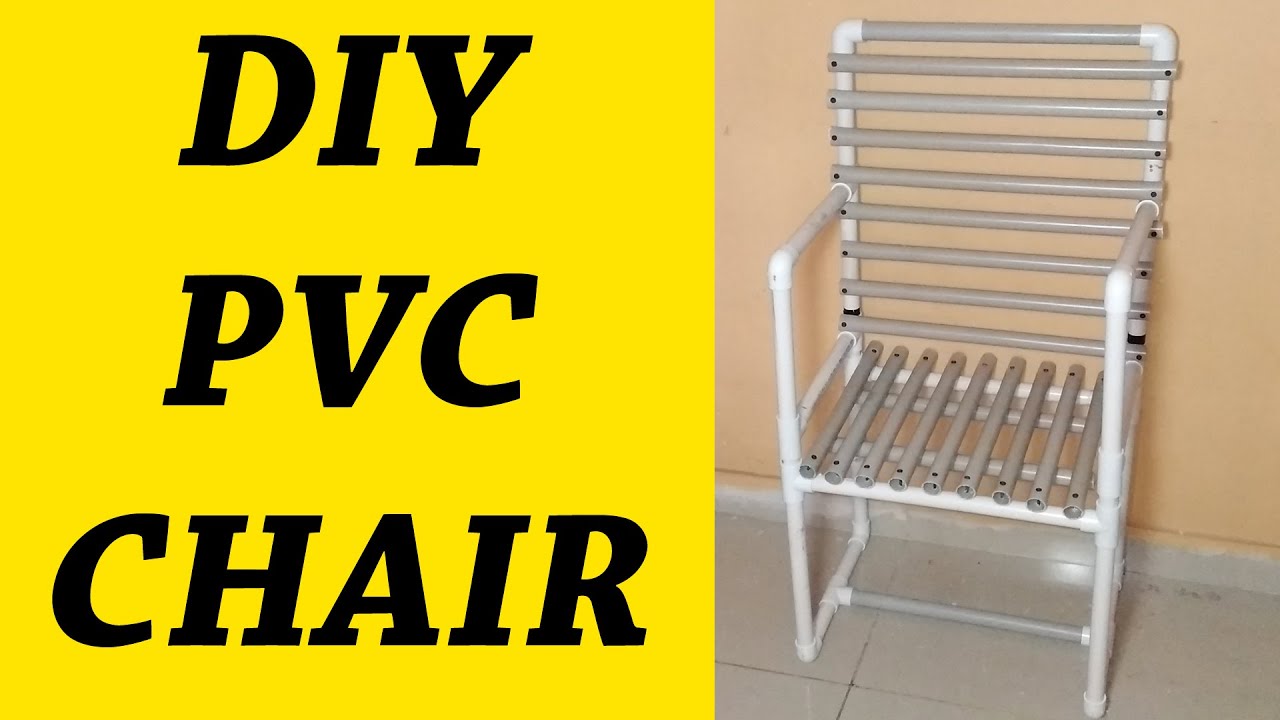The image is a rectangular, color photograph in landscape orientation, measuring about six inches wide and three inches high. The image is divided into two sections with the left side slightly wider than the right side. The left portion features a golden-yellow background with three lines of bold, black text that read: "DIY PVC Chair." On the right side, there is a photographic depiction of an indoor chair made from PVC pipe. 

The right-hand photograph shows a chair with a frame constructed of white PVC pipe, including curved joints. The chair features horizontal gray strapping across the seat and the back. Its frame includes armrests, sides, and vertical slats on the back. The chair appears to have a back and arms, with rectangular frames on the sides connected at the bottom by a horizontal piece of pipe. The setting includes a peach-colored wall with a white baseboard, where some peach paint has slightly overlapped onto it. The floor is covered with light grey tiles.

The image combines elements of photographic realism with graphic design, emphasizing the DIY construction and material details of the PVC chair.